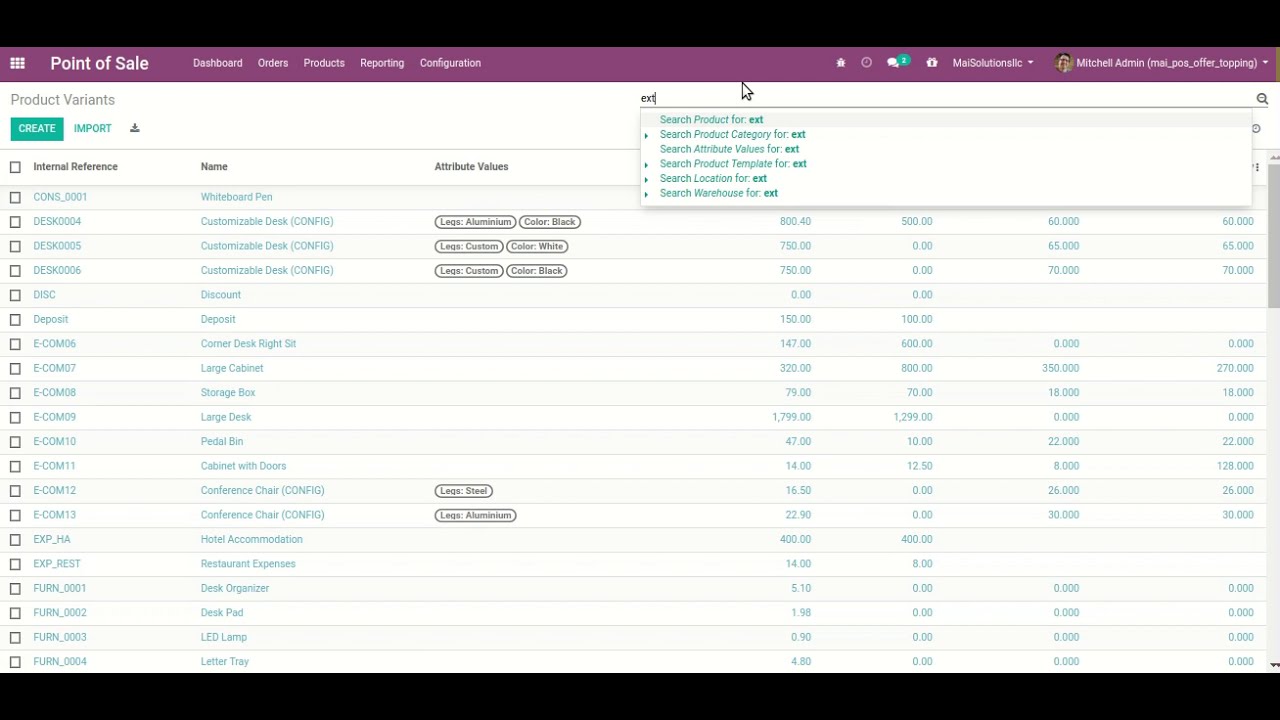The image is a detailed screenshot of a point-of-sale (POS) software application, specifically depicting the interface used for managing invoices. The top left corner prominently displays the heading "Point of Sale," and adjacent to it, there are clickable sections listed as "Dashboard," "Orders," "Products," "Reporting," and "Configuration" within a distinctive magenta banner that spans across the screen. 

On the right side of this banner, user information is displayed, identifying the active user as "Mitchell Admin." The screen shows an interface primarily composed of white background with teal or blue text. A black bar runs along both the top and bottom edges of the image, framing the central workspace.

The primary section of the image contains a list of invoices, each row marked with blue text and a checkbox on the left, allowing for selection. The columns are clearly labeled with headers such as 'Internal Reference,' 'Name,' and 'Attribute Values,' among others. Specific items are listed under 'Name,' including "Deposit," "Large Cabinets," "Storage Box," "Large Desk," "Pedal Bin," "Cabinet with Doors," "Desk Organizer," "Desk Pad," "LED Lamp," and "Letter Tray."

A cursor hovers over a search bar at the top center of the interface, where the user is inputting the letters "EXT," presumably searching for a specific item. This interaction partially obscures some of the data fields below it. Overall, the image conveys a functional and organized POS interface used for managing products and orders within the application software.